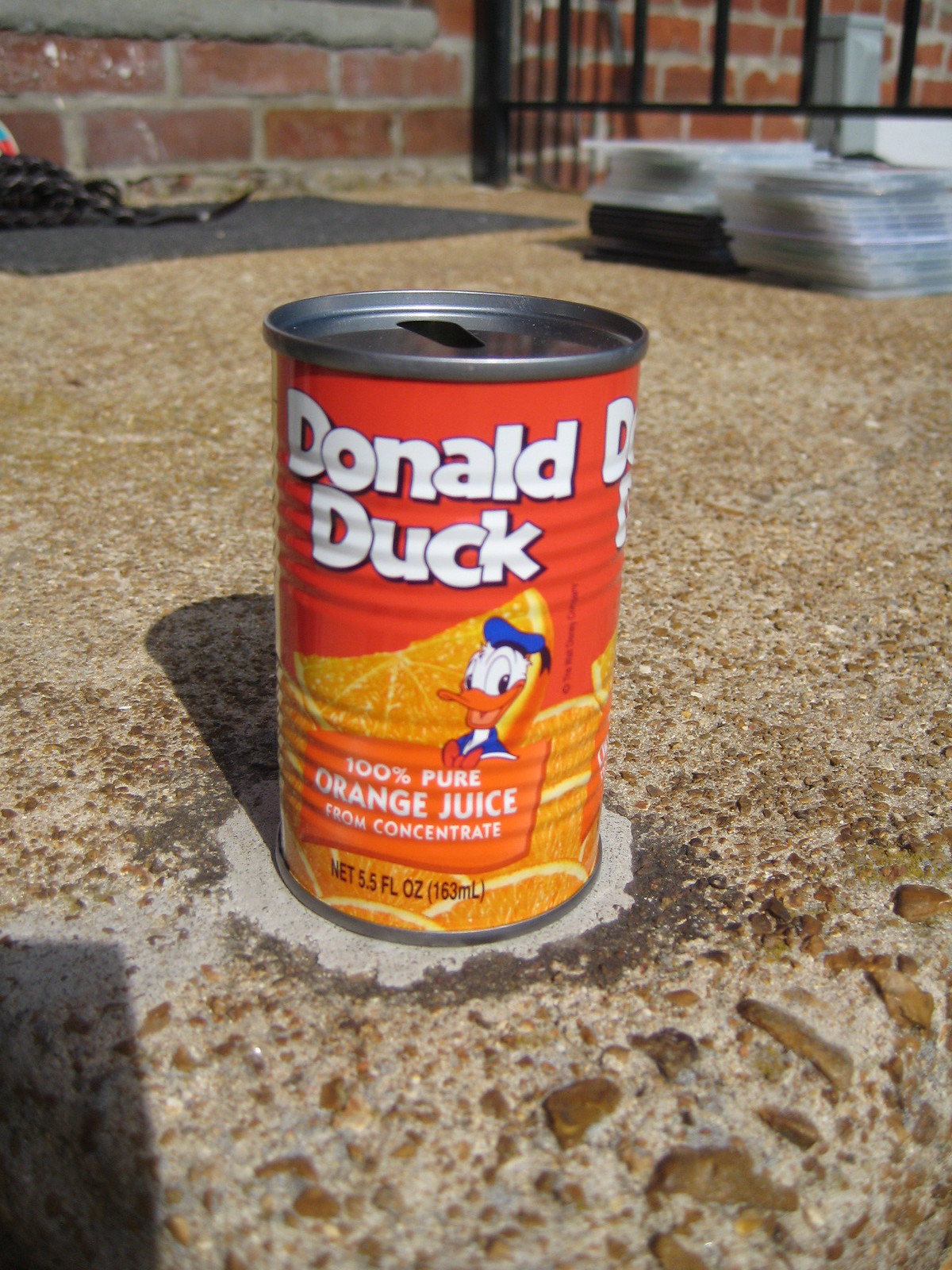A red can labeled "Donald Duck" is prominently displayed on the pavement in front of a brick building. The front of the can features an illustration of the classic Disney character, Donald Duck, who is depicted as a white duck wearing a blue sailor's outfit and hat, with a red bow tie. The text on the can reads "Donald Duck" in white letters, along with "100% Pure Orange Juice From Concentrate." Additionally, decorative orange slices are scattered around the can's design. The text at the bottom of the can indicates the volume as "Net 5.5 Fluid Ounces (163 Milliliters)."